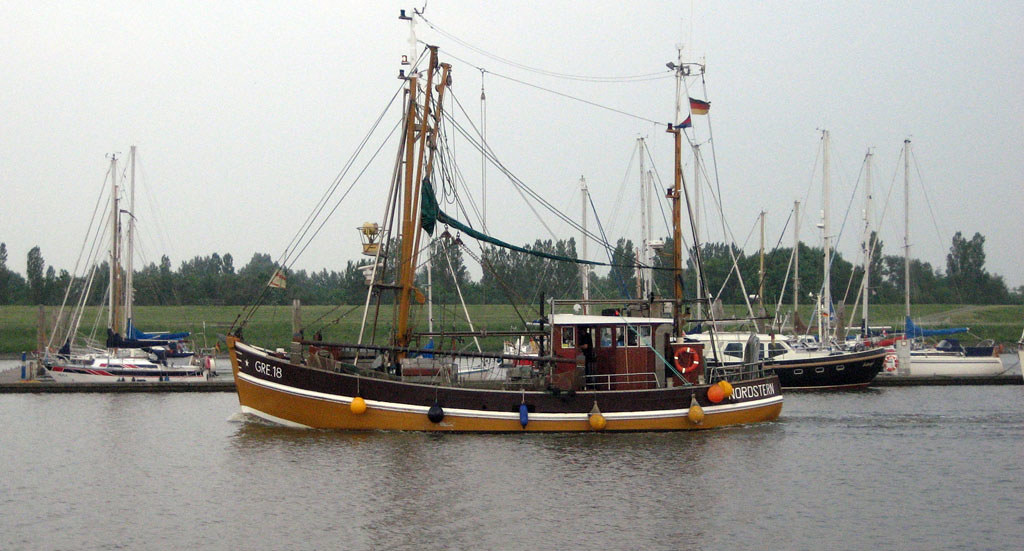This is a color photograph in landscape orientation capturing a serene bay or ocean setting populated with several sailboats. The central focus is a large, orange and brown sailboat named "Nordstern" positioned closest to the viewer, with distinctive red cabin, two large masts, and a visible white roof tower where the operator would sit. The boat features a black section along the top border, followed by a white stripe, and then a brown wood tone stripe. Various floats can be seen hanging over the edge of its rail. To the left of the "Nordstern," there's a red, white, and black sailboat, along with another blue-hued one. On the right, additional boats with numerous visible masts—about nine or ten—are moored or docked behind the central boat, including a black boat with white trim.

The water, displaying a gray-blue tint, reflects the overcast, light blue, and somewhat hazy sky, adding a calm and muted atmosphere to the scene. In the background, there's a grassy field, progressing into a row of tall, dark green trees that span the horizon, enhancing the natural and tranquil essence of the photograph. The overall style reflects photographic representational realism, capturing the detailed and picturesque maritime scenery.